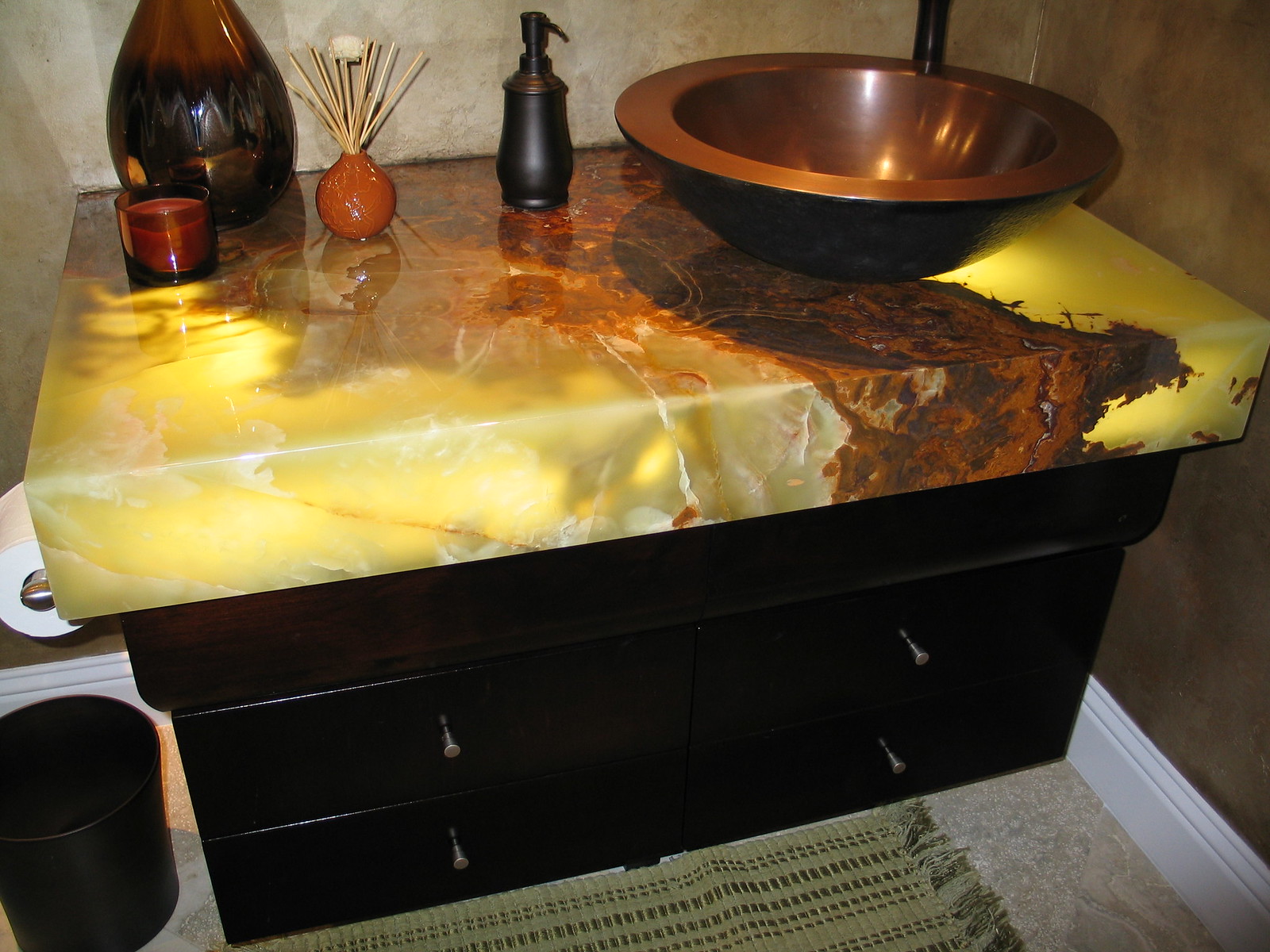This photograph captures an elegant bathroom sink area, dominated by a stunning large rectangular countertop that appears to be crafted from a yellowish stone or marble. The countertop features a striking brown streak that starts at the back and cascades over the front edge, adding a dramatic element to the space. Positioned on the upper right-hand side of the countertop is a distinctive round copper sink, gleaming warmly under the light.

Adjacent to the sink on the left, a sleek black soap dispenser with subtle gold accents stands out. Further to the left, a small vibrant orange vase contains a delicate arrangement of wooden reeds, adding a touch of natural decor. Near this, a larger vase made of transparent brown glass holds its place prominently on the countertop, with a similarly colored small candle placed in front, creating a harmonious color palette.

The base of the counter showcases a rich, dark wood finish, almost black, equipped with four drawers—two on each side—with stylish silver handles providing a touch of modern flair. Below the counter, a gray rug softens the hard surfaces and adds comfort underfoot. To the left of the counter, practical elements such as a roll of toilet paper and a sleek black trash can are conveniently placed, blending function with style in this beautifully designed bathroom space.